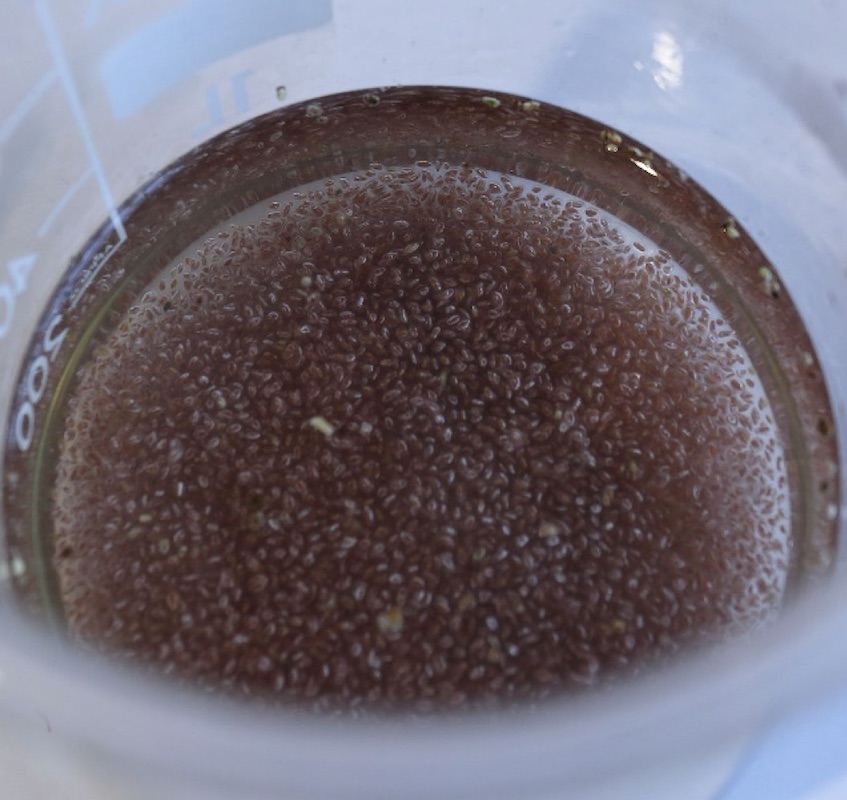This close-up image reveals the inside of a clear measuring cup, specifically focusing on a collection of very small seeds, most resembling black chia seeds, immersed in a liquid that appears similar to almond milk. The liquid shows some light reflections along the upper edges of the cup, which also highlights that the nearest edge is slightly out of focus. The seeds rest at the bottom, predominantly black or dark brown with a few lighter ones dispersed throughout. Visible on the left side of the cup are reversed measurement markings, with the number "200" clearly distinguishable. The detailed close-up perspective provides an intimate look at the seeds soaking in the creamy substance, suggesting a preparation process.